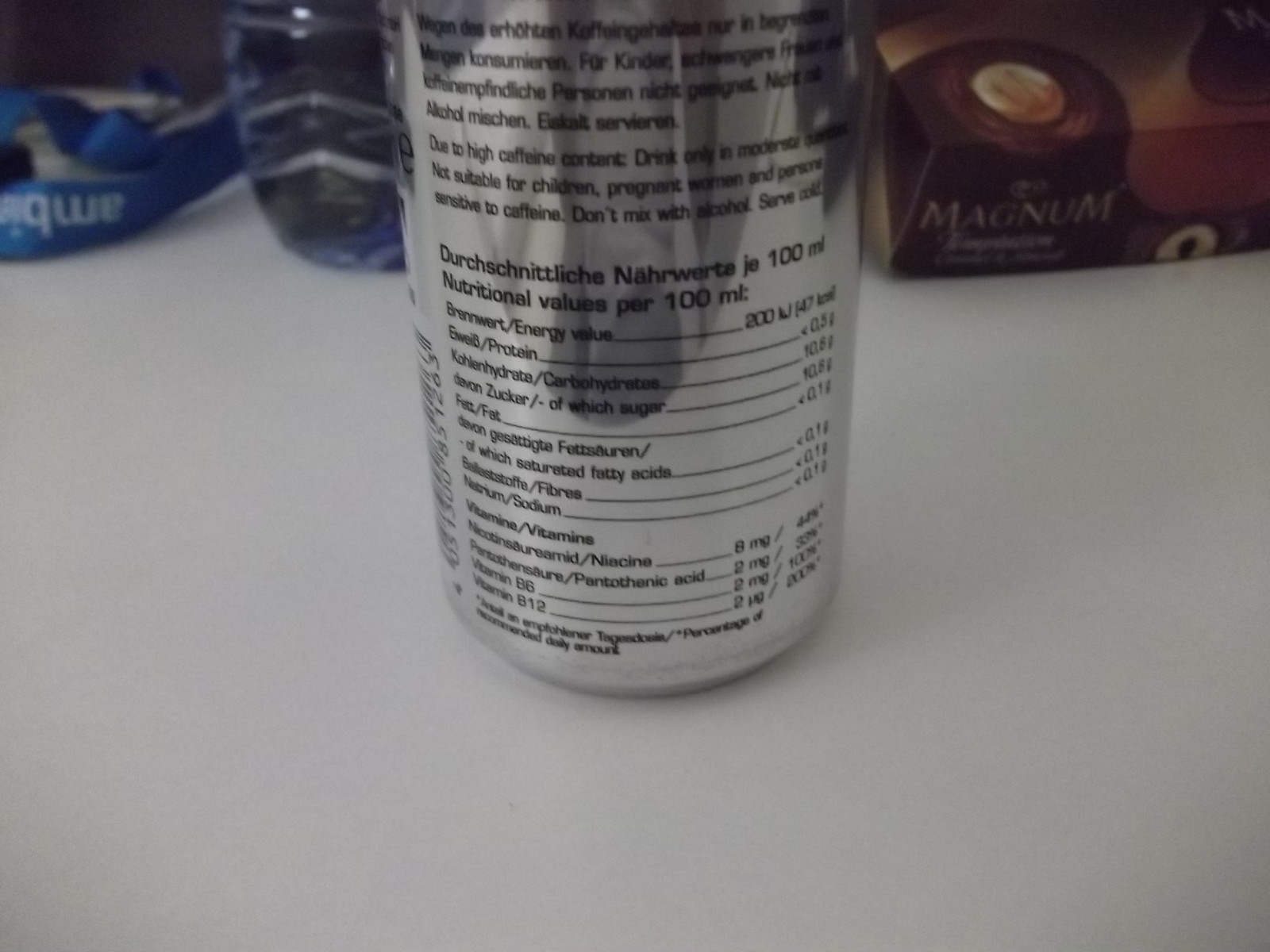This is a color photograph predominantly showcasing a highly reflective aluminum beverage can, positioned centrally on a greyish surface. The can, with its mirror-finish silver exterior, features black text that predominantly lists nutritional information. The text appears in German, followed by an English translation, detailing nutritional values per 100 milliliters. The left side lists various ingredients, while the right side specifies their quantities.

In the background, there is a line of objects partly visible, including what seems to be a blue strap with some white writing on it, and a glass containing some form of liquid on the left. On the right side, a box of Magnum chocolate, characterized by its brown color palette, is partially in view. The box depicts a Magnum chocolate bar with a brown exterior and a cream filling, along with the brand name written underneath the image.